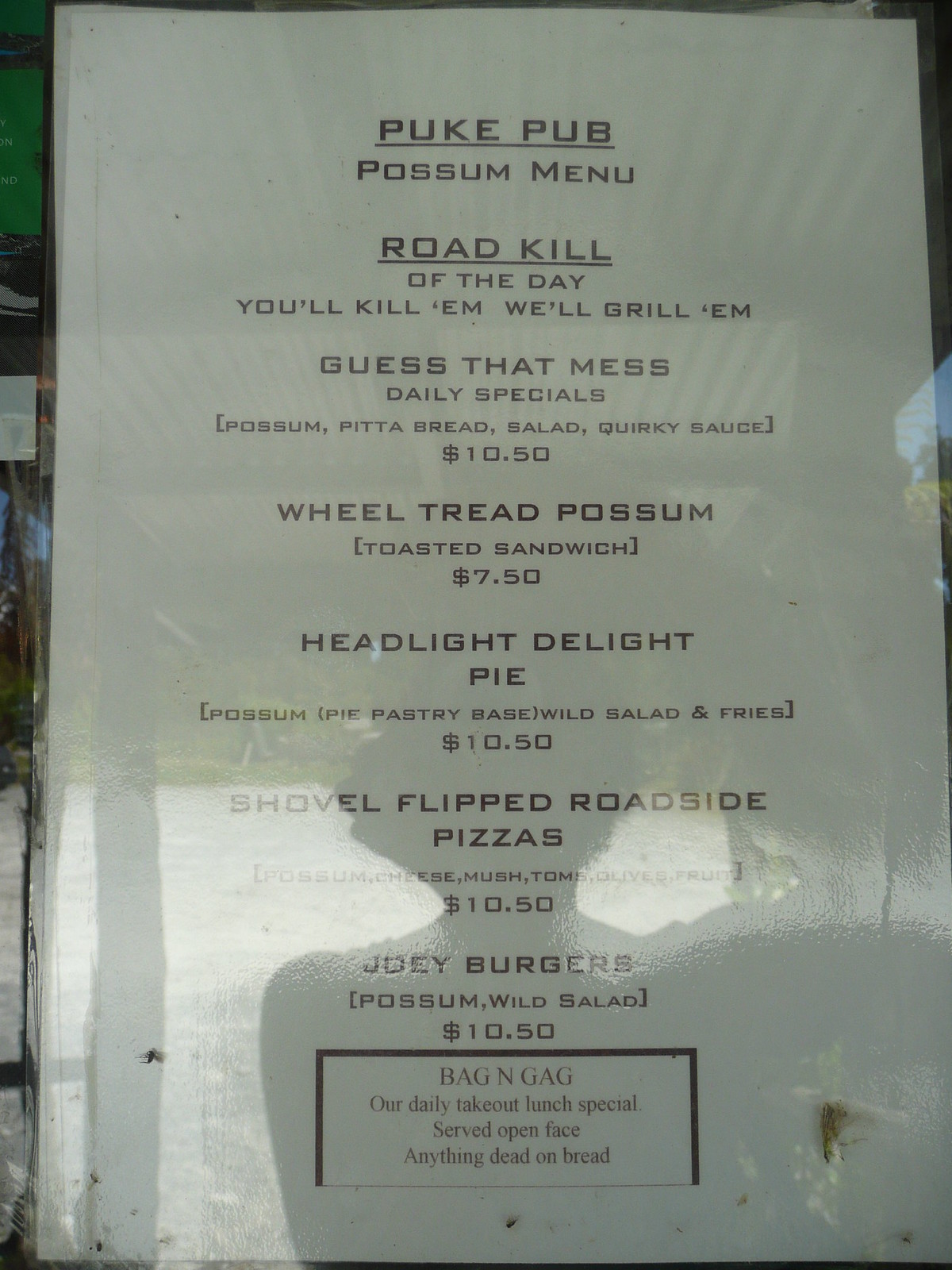The image depicts a full-sized black-and-white menu posted on a glass window, through which a person's silhouetted reflection and bright light can be seen. The establishment is named "Puke Pub," which is prominently displayed at the top of the menu. Below the title, a horizontal line separates it from the subheading "Possum Menu." 

The menu's theme centers around roadkill cuisine, with the phrase "Roadkill of the day" followed by the peculiar slogan "You kill him, we'll grill him." Another section called "Guess That Mess" lists daily specials, all featuring possum meat. These offerings include possum served with pita bread, as a sandwich, in a pie, on a pizza, and as a burger. 

At the bottom of the menu, the "Bag and Gag" section advertises the daily takeout lunch special, whimsically described as "served open-face, anything dead on bread." While it's uncertain if the menu is genuine, the playful and macabre descriptions certainly catch the eye.